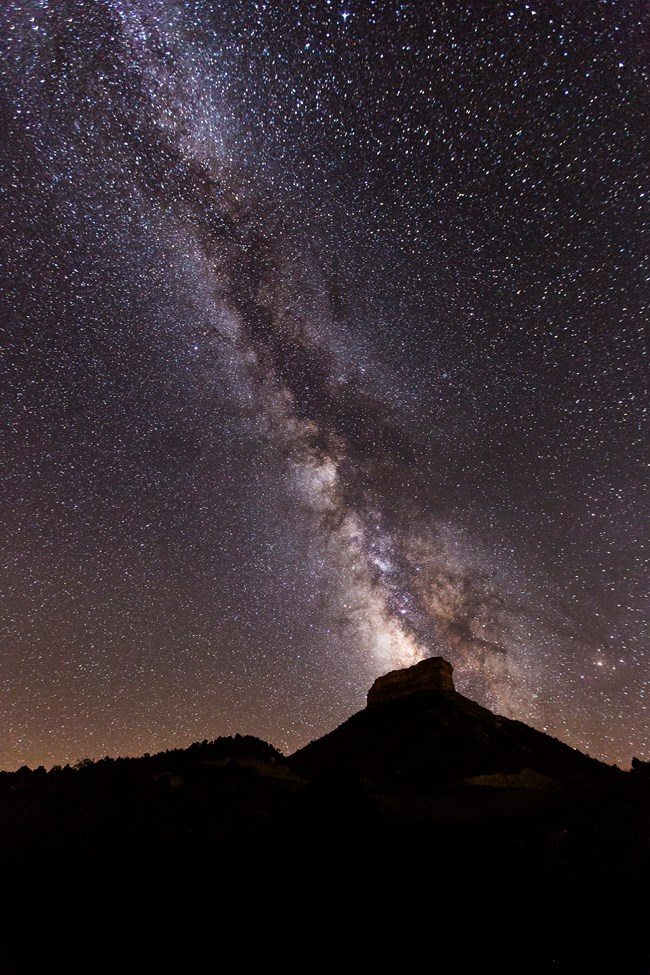This image captures a stunning night scene dominated by the celestial beauty of the Milky Way, cutting a striking path through the center of the photograph. The vast night sky, taking up about 80% of the frame, is a profound black canvas peppered with countless white stars. The Milky Way extends diagonally from the top left to the bottom right, with its brightness diminishing towards the right. The left side of the Milky Way glows brightly, contrasting with the fainter right side. The stellar display ranges from dark purples to light purples and soft pinks, enhancing the vivid nightscape.

In the completely dark foreground, a silhouetted mountain with a distinctive boxy summit sits as a prominent feature. This mountain appears like a box perched on a triangular base, providing an interesting geometric contrast against the endless sky. Adjacent to the mountain, a tree-lined hill emerges to the left, its outline faintly visible. The entire foreground, whilst almost black, hints at the rugged terrain below, likely a plateau or mesa set in a desolate landscape. The interplay of these natural elements with the dazzling night sky creates a captivating and detailed nocturnal scene.